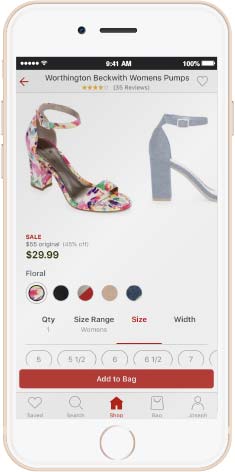The image depicts a highly detailed and clean screenshot of someone's phone, showing an online shopping interface for shoes. The phone is encased in a housing that appears to be either a salmon pink or a creamy vanilla white. 

The screen is white, featuring a central off-white section dedicated to an advertisement. At the top of this section, a horizontal black bar displays the current time (9:41 a.m.) and the phone's battery status (100%). Below this bar, the advertisement details "Worthington Beckwith Women's Pumps," rated four out of five stars. On the left side, there is an image of a floral-adorned, open-toe, ankle-strap, chunky heel shoe. To the right, a gray silhouette of the same shoe illustrates its shape without any decorative elements.

Highlighted in red text, the advertisement notes that the shoes are on sale for $29.99, reduced from their original price of $55. The text also mentions that the shoe is available in five different colors, with the floral design being currently selected. Other available colors include black, red and gray, white and gray.

Below this, there is an interface for selecting the quantity, with the current quantity set to one. The size range is specified for women's sizes, and the user is in the process of selecting their size. A prominent red "Add to Bag" button is available for completing the purchase. 

At the bottom of the screen, a series of navigation icons are visible, including a heart for favorites, a magnifying glass for search, a house for the home page, a shopping bag, and a profile icon for user account management.